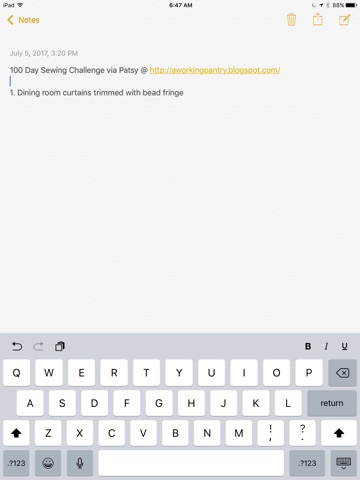This is a detailed screenshot taken from an iPad, displayed in a portrait orientation with approximately a 2:1 height-to-width ratio. The background is gray. The visible on-screen keyboard at the bottom also has a gray background, white keys, and black lettering.

At the top of the screen, in black font, the word "iPad" is displayed on the left, next to a fully filled Wi-Fi symbol. The time "6:47 AM" is centered. To the right of the time, there is a series of icons: a moon symbol indicating 'Do Not Disturb' mode, a navigation arrow pointing upwards and to the right, a Bluetooth icon, and finally, an 88% battery status indicator next to a black nearly full horizontal battery icon.

Below the status bar, an orange left-facing arrow and the word "Notes" are displayed on the left. To the right of these are a trash can icon, an upload icon, and an edit button. Just beneath this toolbar, the text "July 5, 2017, 3:20 PM" appears in a light gray font.

The main body of the screenshot contains black text reading: "100 Day Sewing Challenge via Patsy at" and then an orange hyperlink "working pantry dot blogspot dot com." This is immediately followed by a blue cursor. Below the cursor, another line of black text reads: "One dining room curtains trend with bead fringe."

The remainder of the screen beneath this text is primarily white or gray space, leading down to the aforementioned on-screen keyboard.